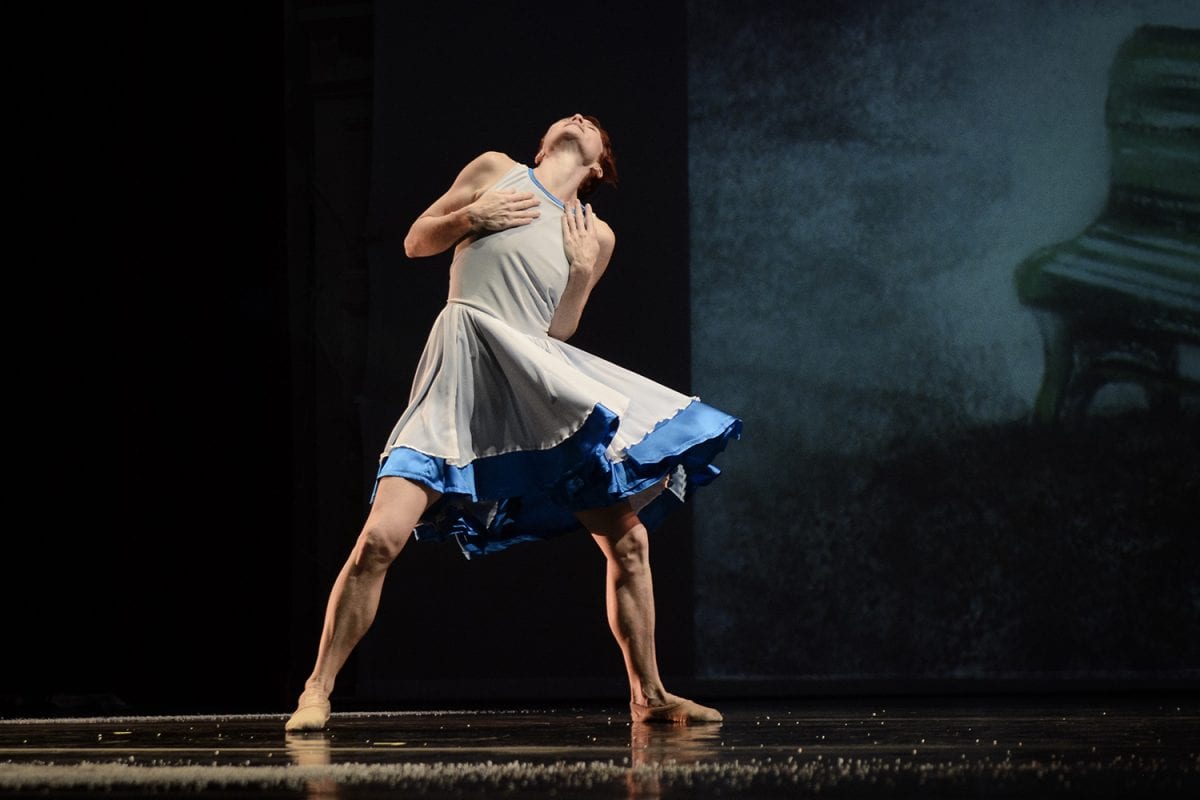The image portrays a dynamic action shot of a dancer performing on a dark stage. The backdrop is predominantly black with a sketch of a bench visible on the right side, extending vertically from the floor to the ceiling. The dancer, who appears to be performing a ballet, is captured mid-movement with their head thrown back and hands pressed to their chest. They are barefoot and dressed in a white skirt with a blue underskirt, and a matching white tank top with blue edging around the neck. While the dancer has muscular features and some characteristics traditionally associated with a male, such as a visible Adam's apple and hints of facial hair, their graceful and elegant movements suggest the expertise of a seasoned ballerina. The floor beneath them is sprinkled with white flecks, adding to the overall ethereal atmosphere of the scene.